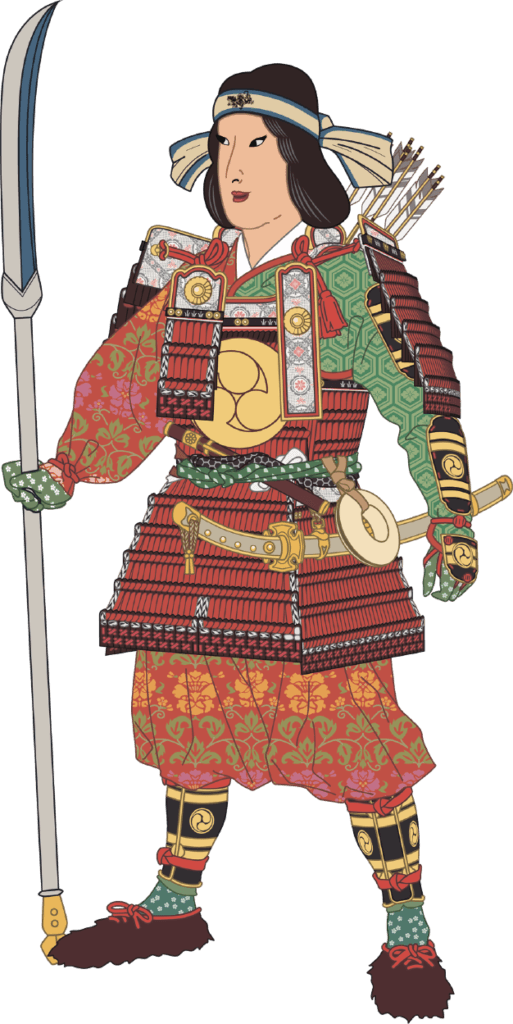This image depicts a striking woodblock-style illustration of a formidable female samurai. She has long, flowing black hair adorned with a white headband, which bears an inscription in black on her forehead. Her lips are painted a vivid red, adding to her fierce appearance. She is garbed in a vibrant, flower-patterned kimono predominantly featuring shades of red, with accents of green and pink. 

Hanging at her hip is a beautifully crafted sword, encased in a white scabbard embellished with gold accents. The hilt of this weapon is also white with matching gold detailing. Tucked into her twisted green waist sash is a mysterious tube. The sash wraps securely around her torso, adding an extra layer of intrigue.

The samurai sports brown shoes laced in red and black shin pads adorned with an emblem, indicating perhaps her clan or status. In her hands, she wields a naginata, a traditional Japanese pole weapon, with a gray pole and a blade that features a section of blue, alongside a golden base. 

Furthermore, a white circular disc of unknown purpose is fastened to her attire, adding to the enigmatic nature of the character. On her back, she carries a quiver, suggesting she is as proficient with a bow as she is with her close-combat weapons, completing her arsenal and underscoring her readiness for battle.